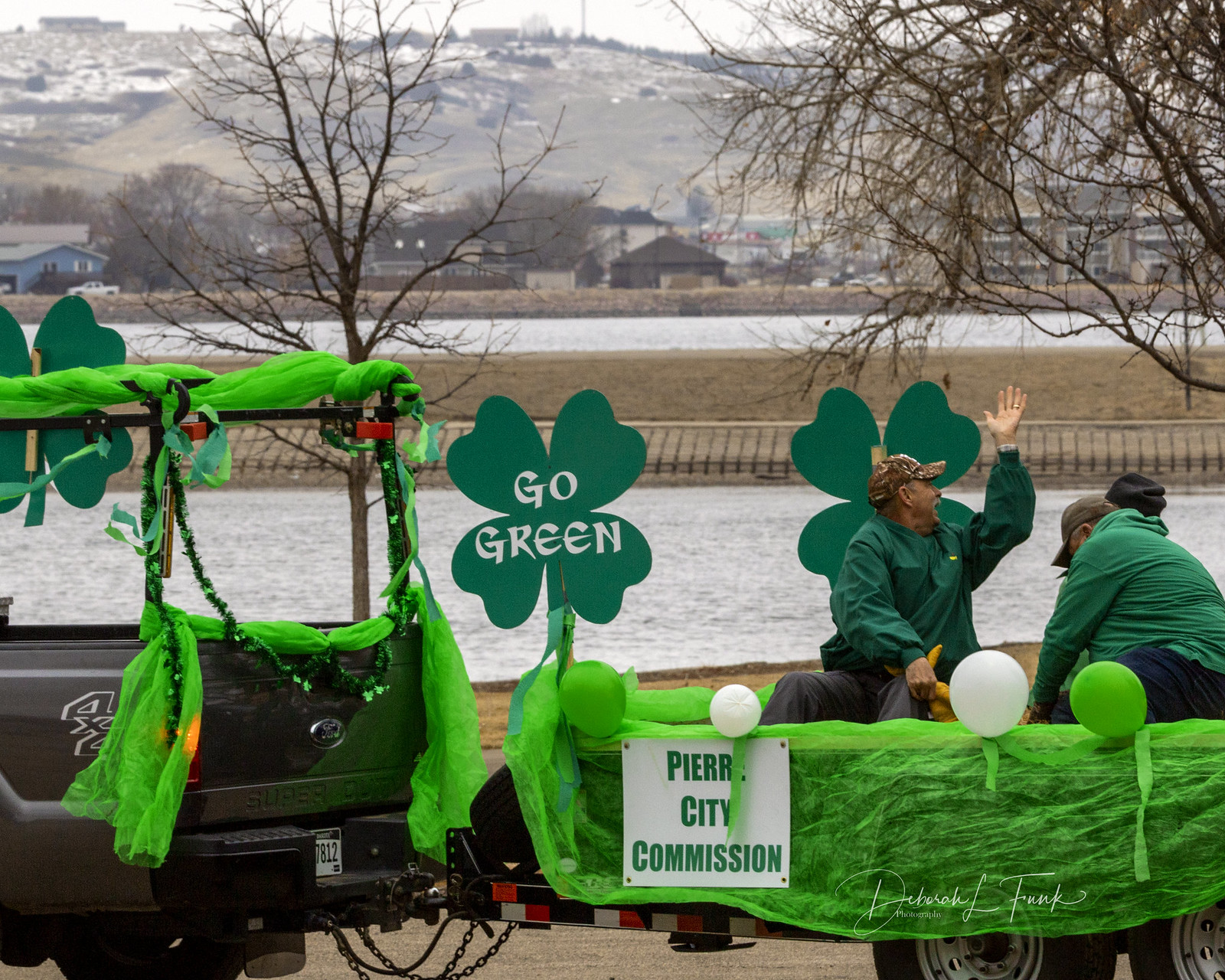The image depicts a St. Patrick's Day parade float, set against the backdrop of a small town with rolling hills, trees, and several waterways. Central to the image is a greenish-gray Ford 4x4 truck, displaying a barely visible license plate, which is pulling a festively decorated trailer. The trailer, associated with the Pier City Commission, is adorned with vibrant green cloth, green and white balloons, and various four-leaf clovers emblazoned with the slogan "Go Green." Two men in green jackets can be seen on the float, waving to the crowd, with bags that might be filled with candy underneath them. In the distance, homes and other buildings can be seen nestled in between the hills. The overall scene captures the festive and communal spirit of the St. Patrick's Day celebration.